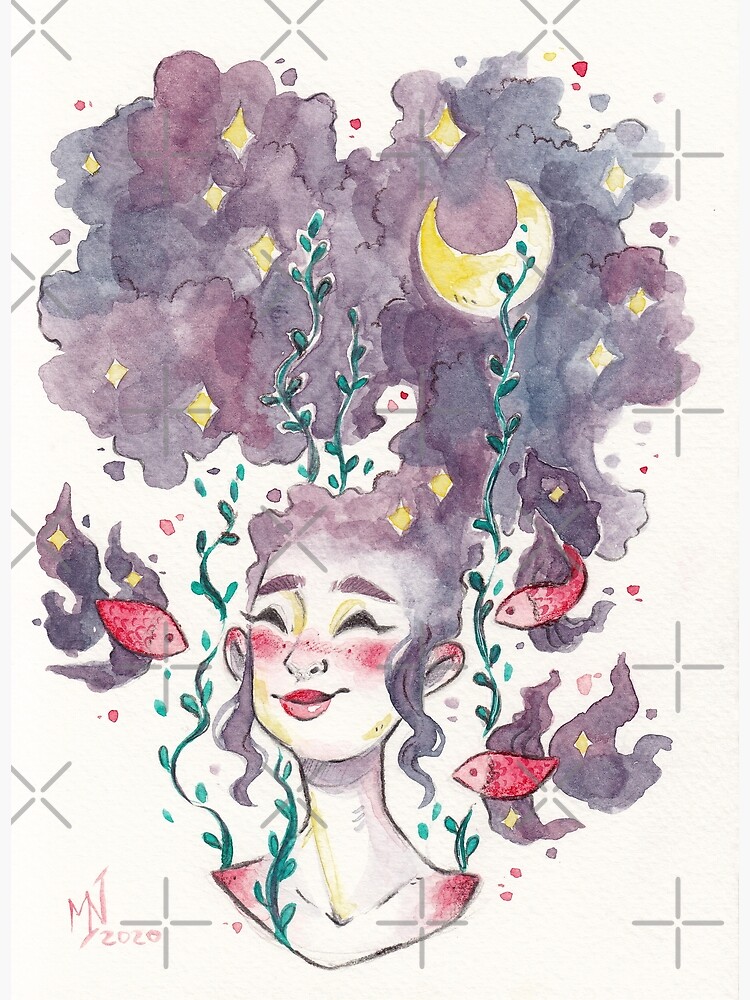In the lower center of the image stands a smiling young girl with curly hair, her eyes closed, and a visage both mysterious and whimsical. The watercolor painting captures only from just below her neck upwards, featuring her red lips, closed eyelids which are black, and purple eyebrows. Surrounding her head, her hair transforms into a swirling purple and black cloud, which holds a vibrant yellow, upside-down moon and several stars. The fantastical scene is enriched by curling green vines that ascend around her and includes three red fish—one to her left and two to her right, blending seamlessly into the red accents on her face and clothing. The background is primarily white, punctuated with a cross pattern of gray pluses and Xs. The bottom left corner of the image is marked "MN 2020," further grounding this ethereal portrayal in a specific moment in time.